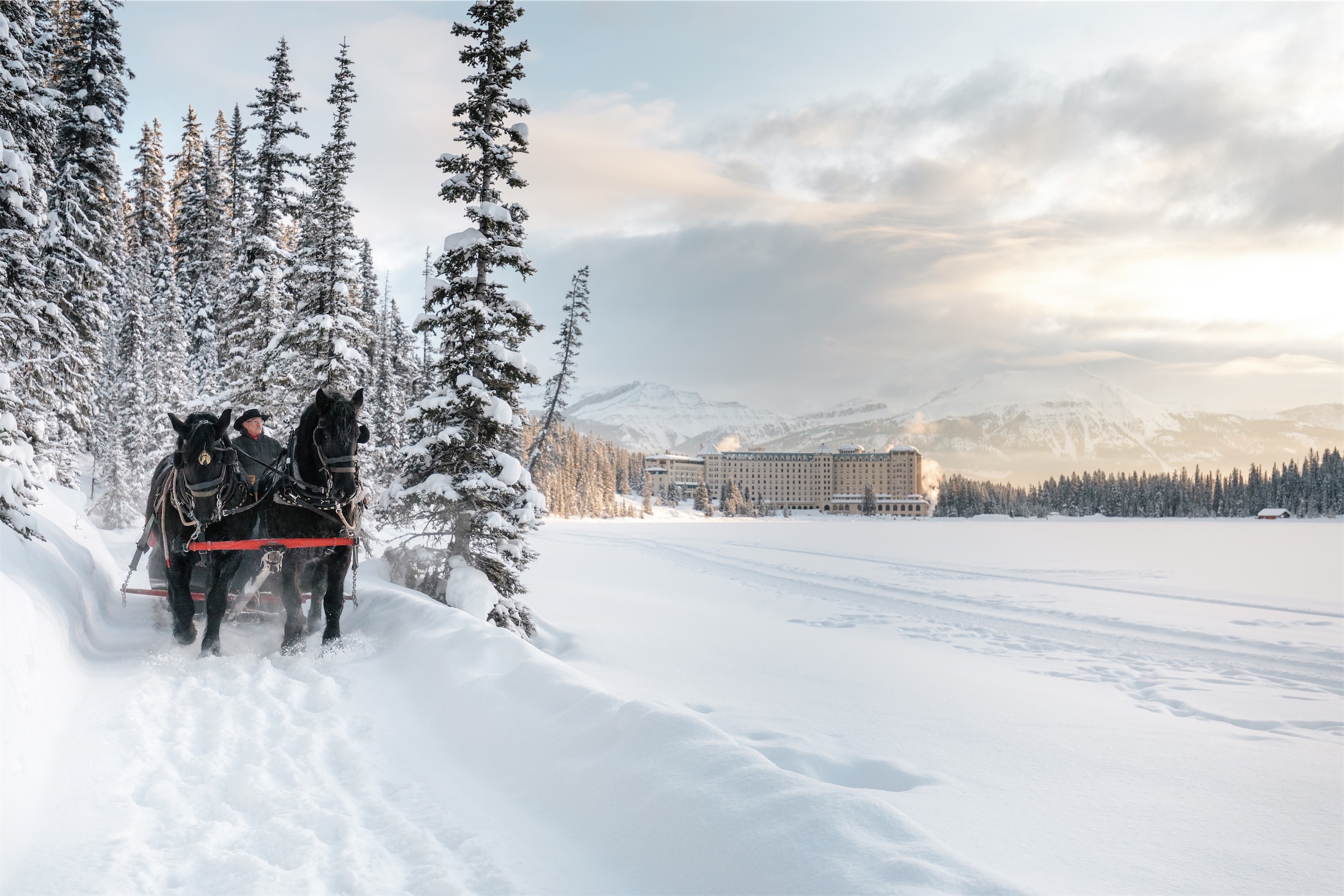In this photograph, the wintry landscape is dominated by a blanket of pristine snow that stretches from the immediate foreground to the distant background. On one side of the scene, two dark-colored horses are prominently featured, each adorned with blinders and accompanied by a somewhat rusted, red metal bar connecting them. These horses are in motion, their powerful legs kicking up a flurry of glistening snow powder as they gallop through the snowy terrain. 

To the side of the horses, a person dressed in a black hat and a black coat holds their reins, expertly guiding them through the snow. The background showcases an array of snow-laden, greenish-hued trees, with some trees displaying a striking yellowish tint and others a darker, denser shade. 

Adding to the picturesque panorama, a tan-colored building emerges in the middle distance. Beyond it, majestic snow-covered mountains rise, their peaks shrouded by a layer of gray clouds that transition into a gray-blue sky overhead. The entire scene captures the essence of a serene, snowy wilderness, infused with the movement and energy of the galloping horses.